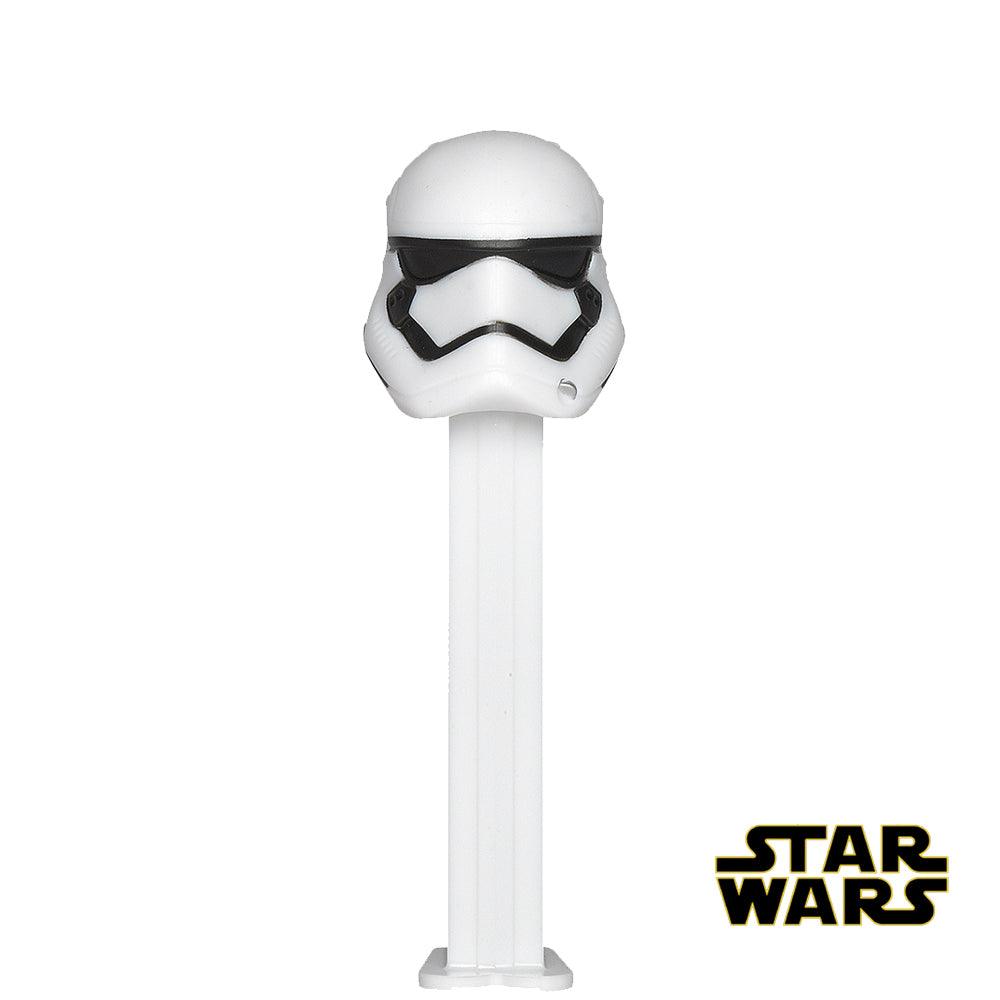The image is a color photograph of a promotional PEZ dispenser from the PEZ candy brand. The dispenser features a classic stormtrooper helmet from the Star Wars franchise at the top. The helmet is white with the distinctive black v-shaped visor, black stripe detailing, and black goggles, characteristic of a stormtrooper's look. The dispenser itself is solid white, with a flat foot base and a long, rectangular, pillared column that leads up to the helmet. Positioned to the bottom right of the image, there is a Star Wars logo in its traditional font, with the word "Star" above "Wars", both outlined in yellow and written in black. The background is bright white, highlighting the white and black colors of the PEZ dispenser, and providing a clean, uncluttered look to the image.